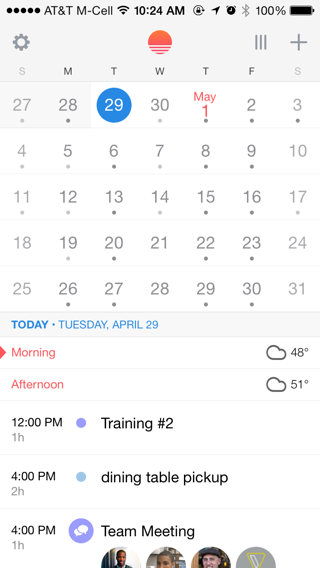This is a detailed photo of an event-tracking calendar in portrait orientation. At the very top, the calendar features a gray border running horizontally across the screen, housing several icons. From left to right, there are five filled dots, an "AT&T" label, the text "M-Cell," a fully filled Wi-Fi signal icon, the time "10:24 AM," a lock icon, a navigation arrow, an alarm clock icon, a Bluetooth symbol, and a vertical battery icon displaying a full charge at 100%.

Below this icon bar, there is a gear icon representing settings, followed by an orange sun-like icon with lines beneath it, and additional buttons to the right. The main calendar section displays the transition from the end of April to the beginning of May. Notably, May 1st is highlighted in orange, indicating it as a significant date. Additionally, Tuesday, April 29th is circled in blue with white numbers, while the remaining dates are in gray.

Underneath the calendar, another gray border displays the current date, "Today, Tuesday, April 29th," along with weather icons depicting clouds for both morning and afternoon. The word "Morning" is highlighted with an arrow. Below this, the schedule includes entries for various events at 12:00 PM and 4:00 PM, listing activities such as trainings, dining table pickup, and team meetings.